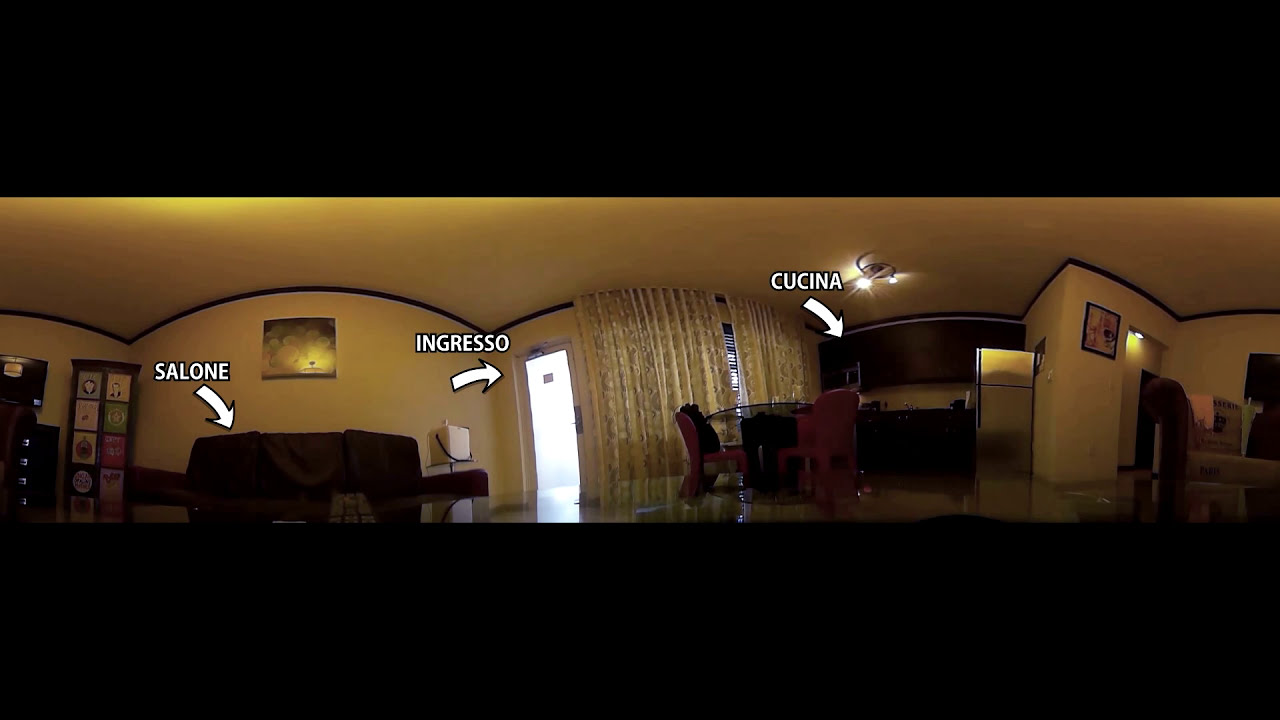This panoramic image depicts the interior of a well-furnished flat or possibly a hotel suite with an open floor plan, labeled with what appear to be Italian words. On the left, the living area is marked as "Salone" and features a dark sofa, a side table with a lamp, a TV on a stand, and a piece of artwork on the wall. The middle section contains a dining area with a table and red leather chairs, leading into a kitchenette labeled "Cucina," which has brown cupboards, a silver fridge, and dark black cabinets with a sink. The walls exhibit a creamy yellow hue, and the floor is a dark brown. The kitchenette is adjoined by a picture-adorned wall and a curved wall section that rhythmically juts out and recedes. To the right is a doorway labeled "Ingresso," suggesting an entrance, possibly leading to the bedroom or bathroom. This doorway floods the room with light and is flanked by a window with curtains. The overall image has a dark yellow cast, bordered by wide black stripes at the top and bottom.